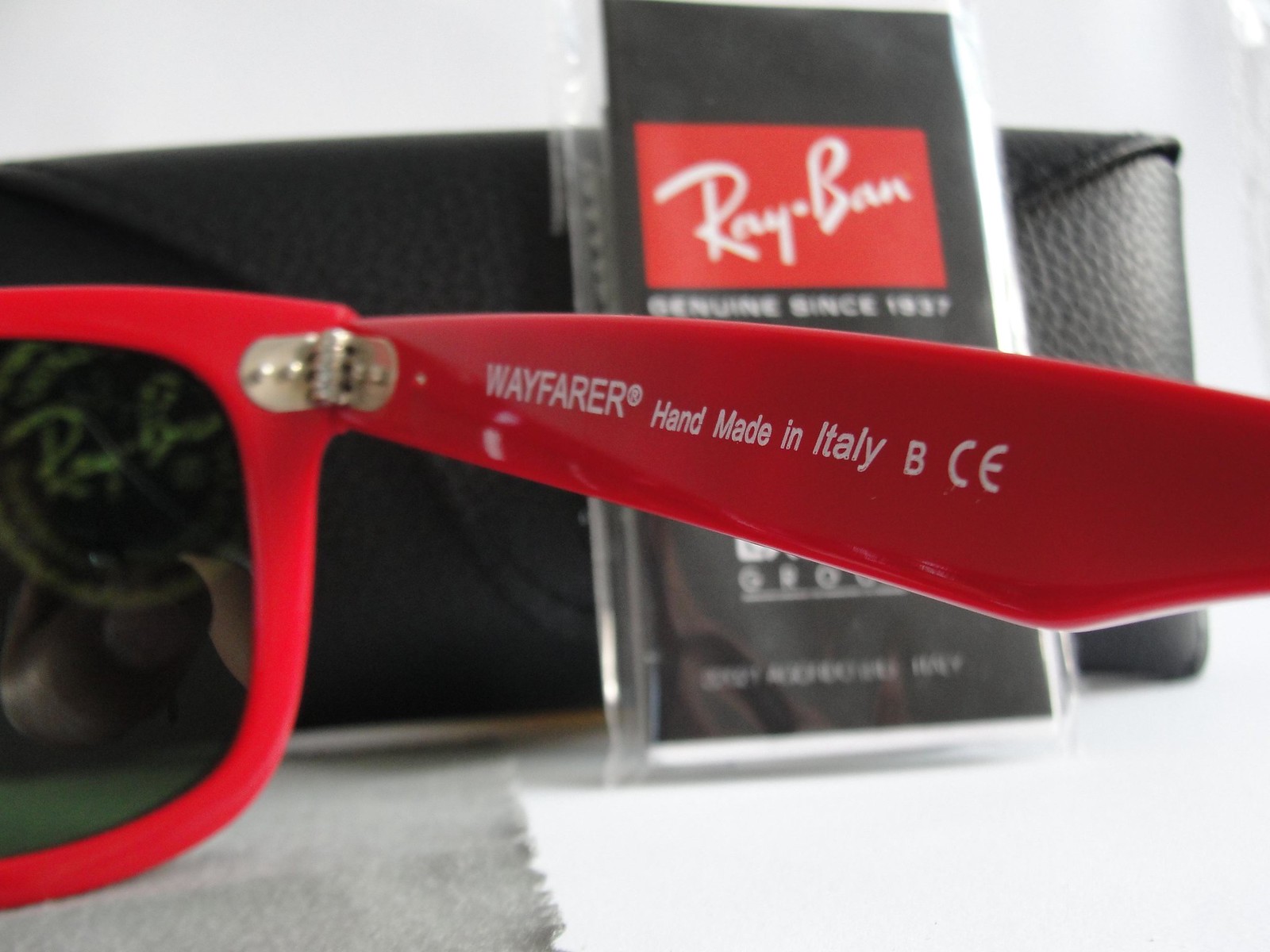The image is a detailed, close-up photograph of the right arm of a pair of bright red-orange Ray-Ban Wayfarer sunglasses. The frame, cut off partially on the left side, prominently displays the white text on the inside reading "Wayfarer, handmade in Italy, B CE." The other details, such as the hinge and the part that rests on the side of the head, are clearly visible. Behind the sunglasses, a black faux leather Ray-Ban glasses case props up a slightly blurred plastic baggie featuring the Ray-Ban logo and a cleaning cloth. Additional text reading "Ray-Ban, genuine since 1937" is discernible on the clear tag. The overall scene is distinct and precisely captured, highlighting both the branding and craftsmanship of the sunglasses and their accessories.